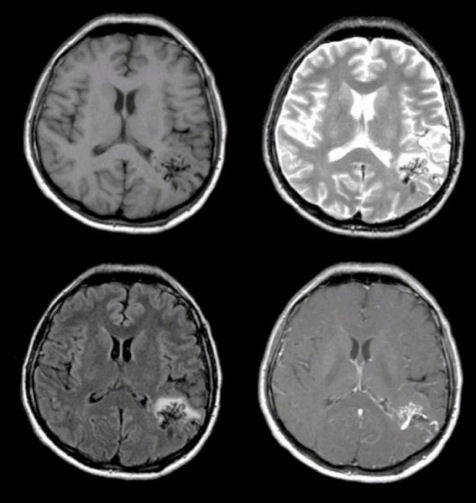The image showcases four distinct MRI cross-sections of a human brain, all against a black background. Each quadrant emphasizes slightly different aspects and contrasts of the same brain. The upper left MRI reveals a brain with a noticeable lesion on the bottom right, the interior predominantly gray with black areas and outlined in white. The upper right section shows the brain with higher contrast, where the lesion and internal structures are more pronounced due to the use of a contrast agent, giving it a whiter appearance with interspersed gray. The lower left image maintains less contrast and highlights the lesion with a white tracer, featuring mainly two shades of darker gray. In the bottom right section, the brain appears mostly as a smoother gray blob, still outlining the lesion albeit less distinctly. Each image, distinguished by varying levels of detail and contrast, provides a comprehensive view of the brain's affected areas, enhancing the understanding of the lesion's presence and structure.